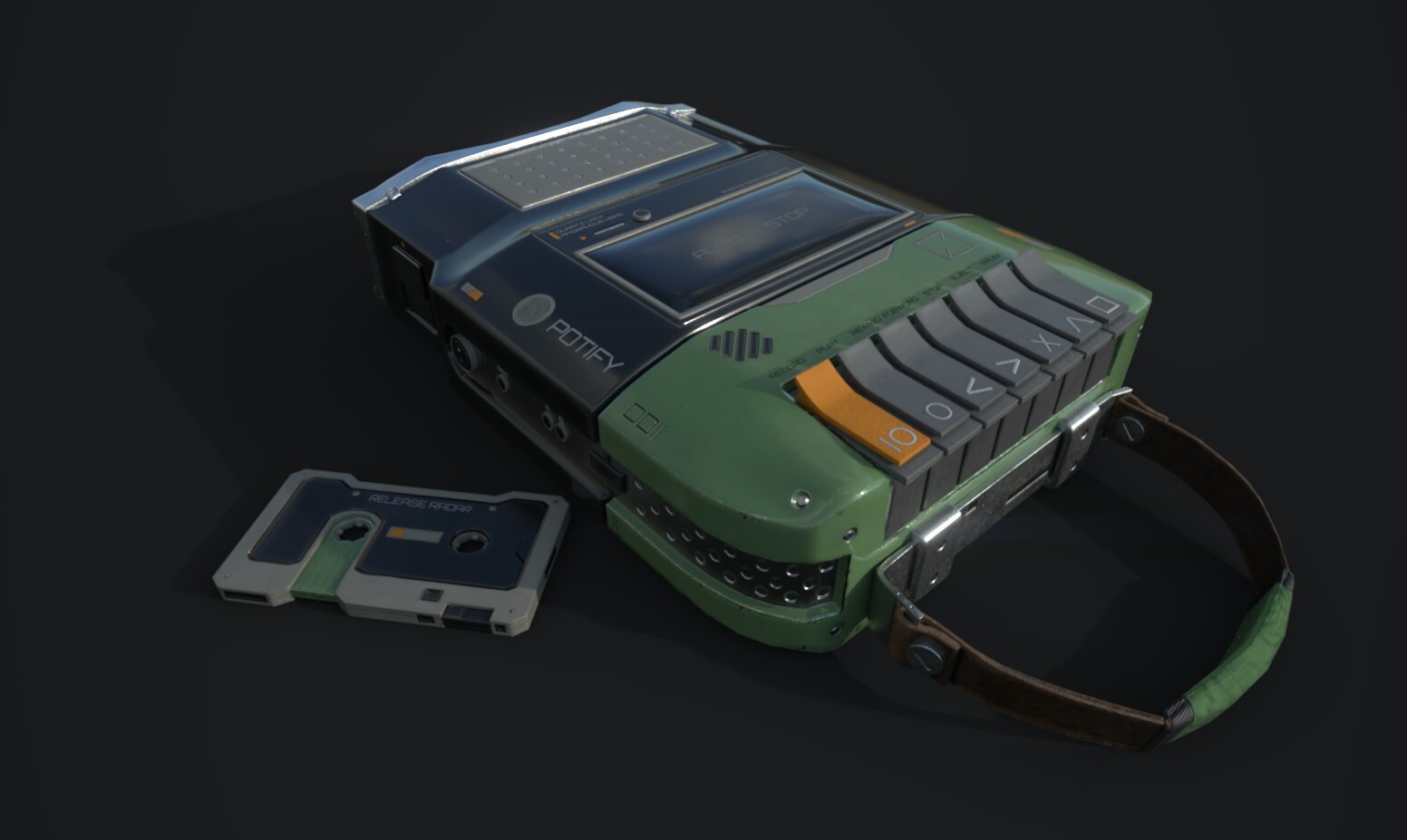This detailed color photograph, set against a black background, prominently features a vintage, green and black tape recorder with the brand name "POTIFY" written vertically on the left side of the tape deck. To the right of the tape recorder is a handle made of brown leather with a green area on top. The cassette recorder is distinctive for its viewing window in the middle and a series of seven buttons situated above the handle. These buttons, which are rectangular and curved upwards, include one orange button marked with the number 10, and six gray buttons with various symbols: a zero, a left-pointing arrow, a right-pointing arrow, an X, an upward-pointing arrow, and a square. Additionally, a white and black cassette tape lies next to the tape recorder, labeled "Release Radar." This image captures the retro aesthetic and unique design elements of the tape recorder and cassette tape, all placed on a featureless black background.